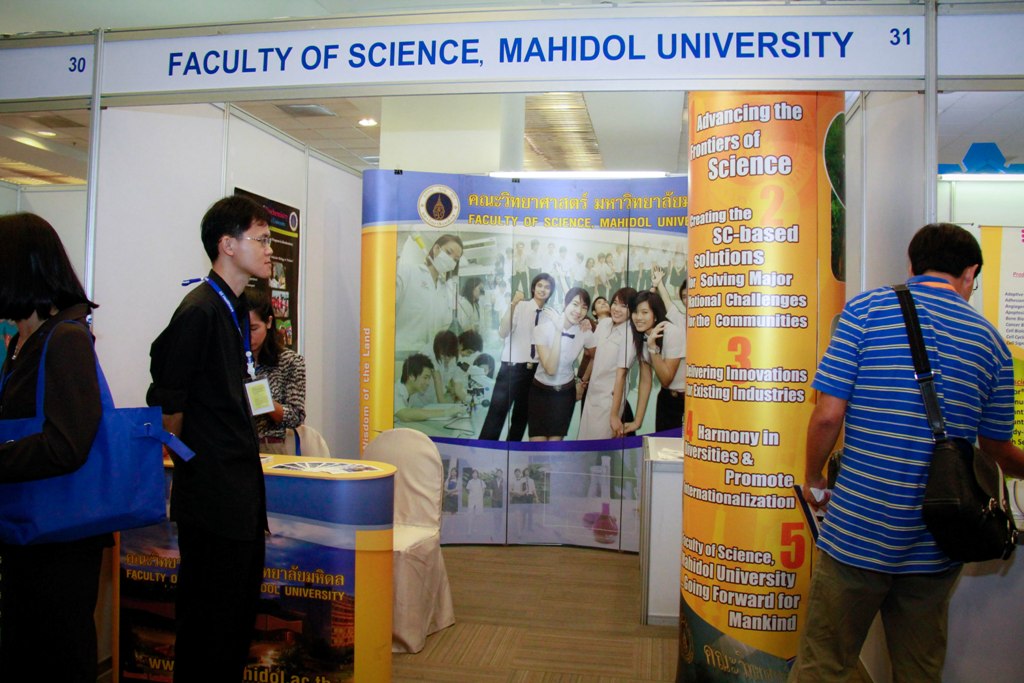The image depicts a bustling booth at a recruiting fair, prominently labeled "Faculty of Science, Mahadol University" in blue letters at the top, with the number 31 underscoring its position. The booth is flanked by adjacent booths numbered 30 and 32, divided by large white panels. Central to the scene is a small counter adorned with a banner, accompanied by two unoccupied chairs behind it, and another counter further back. A series of backdrops and signage, including a yellow and orange banner with white text reading "Advancing the Frontiers of Science, Creating SC-based Solutions, and Solving Major International Challenges for the Communities," adds to the information-rich environment.

In front of the booth, three individuals are engaged with the display. One man, dressed in all black with glasses and a blue lanyard, appears focused on a column wrapped with a detailed poster. Another figure, in a blue and green striped shirt with a bag slung over his shoulder, looks downward near the booth. Additional elements in the background include an array of pamphlets and cards spread out on the table, and pictures of boys and girls huddled and smiling for the camera, adding a welcoming touch to the educational setup. The scene suggests an informative and inviting atmosphere for prospective students or attendees at the event.